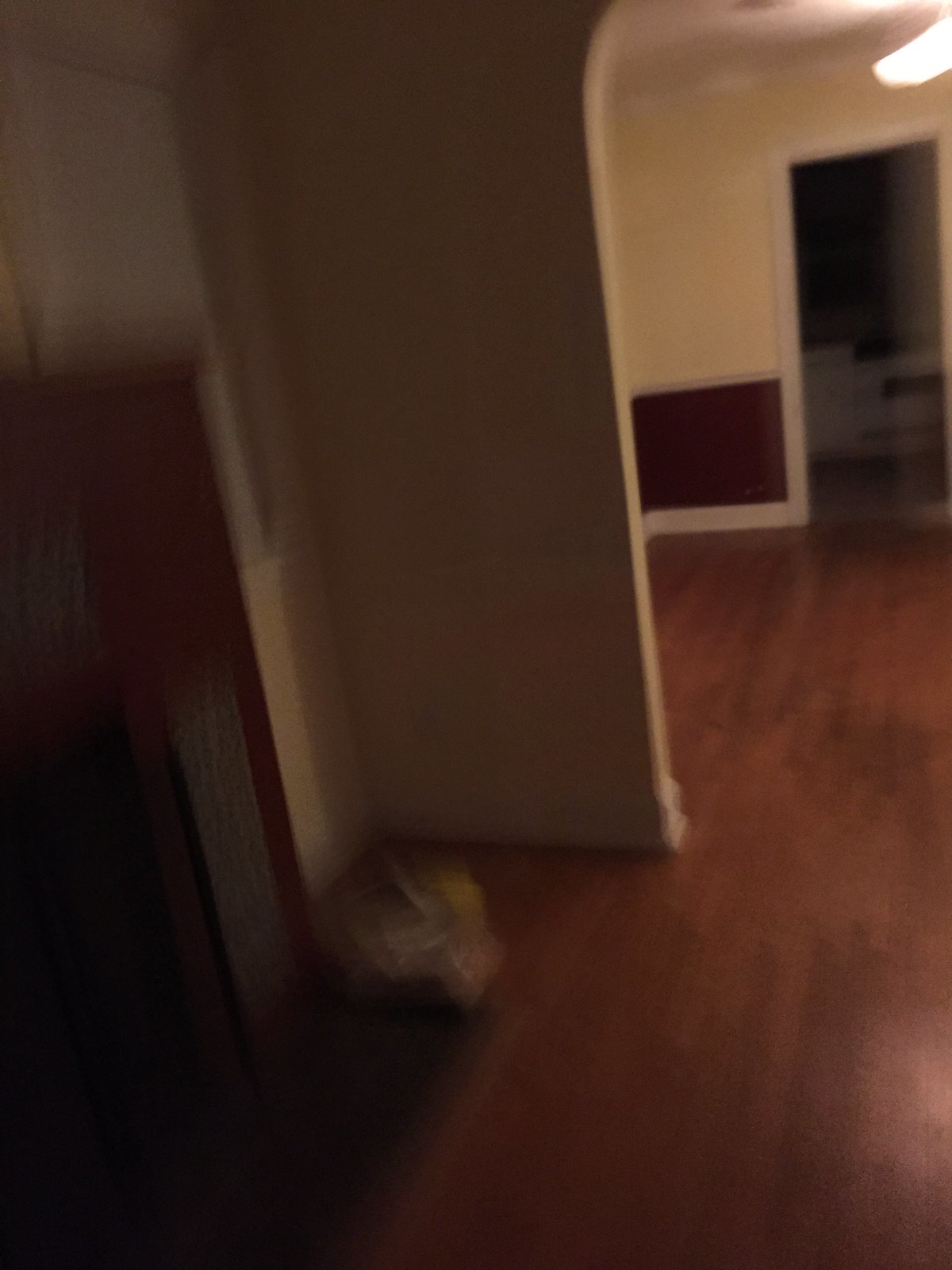The photograph captures the blurred interior of an empty house or apartment. Dominating the foreground is a portion of a dark wood fireplace, set against matching dark wood floors that extend further into the space. Adjacent to the fireplace, a doorway punctuates the wall, providing a glimpse into another room. The room beyond, though blurred, appears to contain counters and lower cabinets, hinting at a kitchen area. In the area closest to the viewer, likely intended as a dining room, the dark wood floor continues, leading up to what seems to be the living room, where the dark wood fireplace is prominently featured.